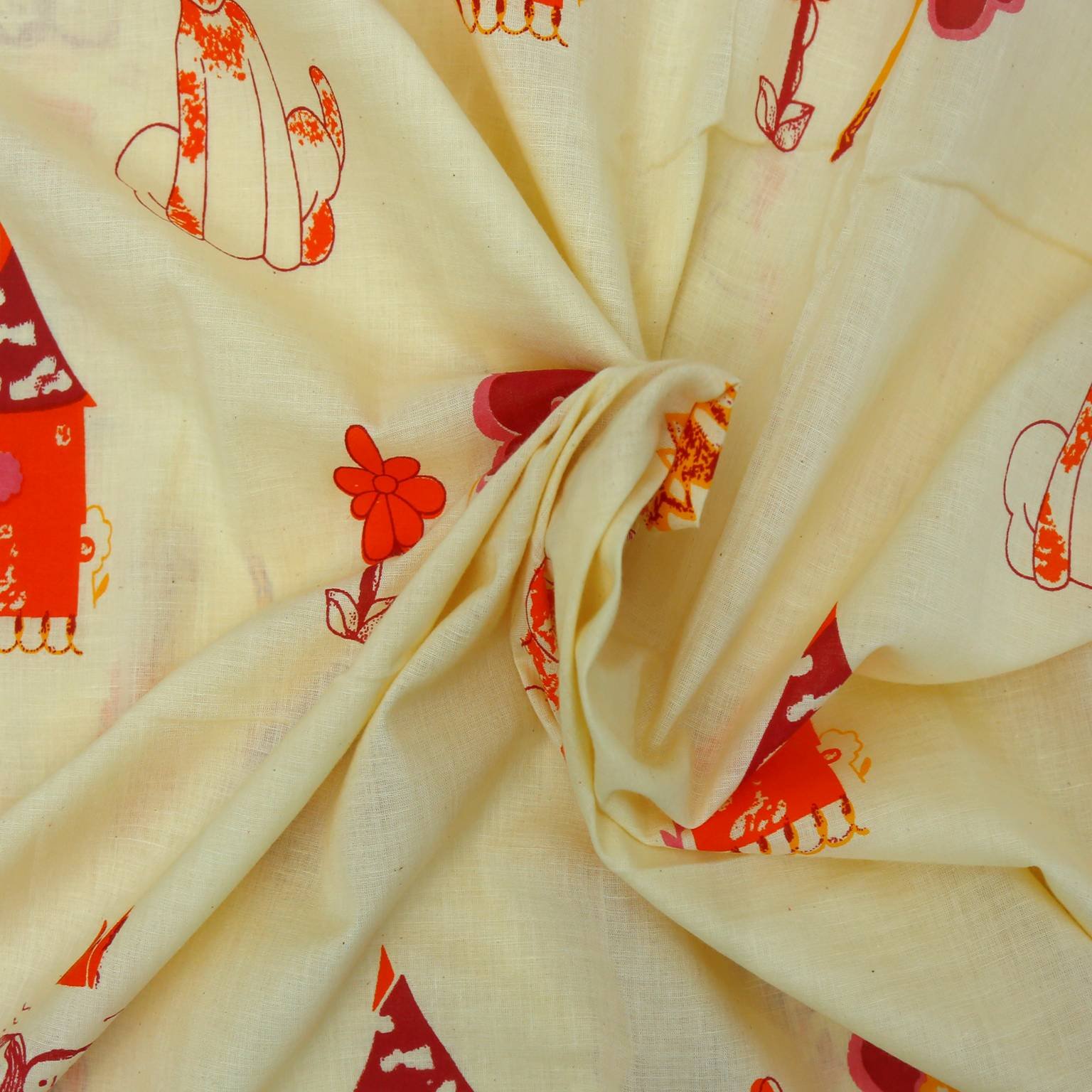This image captures a real-life scene of a piece of lightweight fabric, possibly a blanket, curtain, or scarf. The fabric is predominantly a cream, off-white hue with intricate designs that appear either printed or embroidered. Among the designs are various shades of red, depicting flowers and what seems to be an animal—potentially a cat or dog—partially obscured by the fabric's folds and wrinkles. Scattered across the fabric are multiple objects, including red and orange-red flowers, one with a yellow stem, and what resembles a dog house, reinforcing the likelihood that the animal might be a dog. The fabric is bunched up and twisted in the center, as if someone pinched and turned it, creating a central knot that obscures some of the images and adds a dynamic texture to the scene.